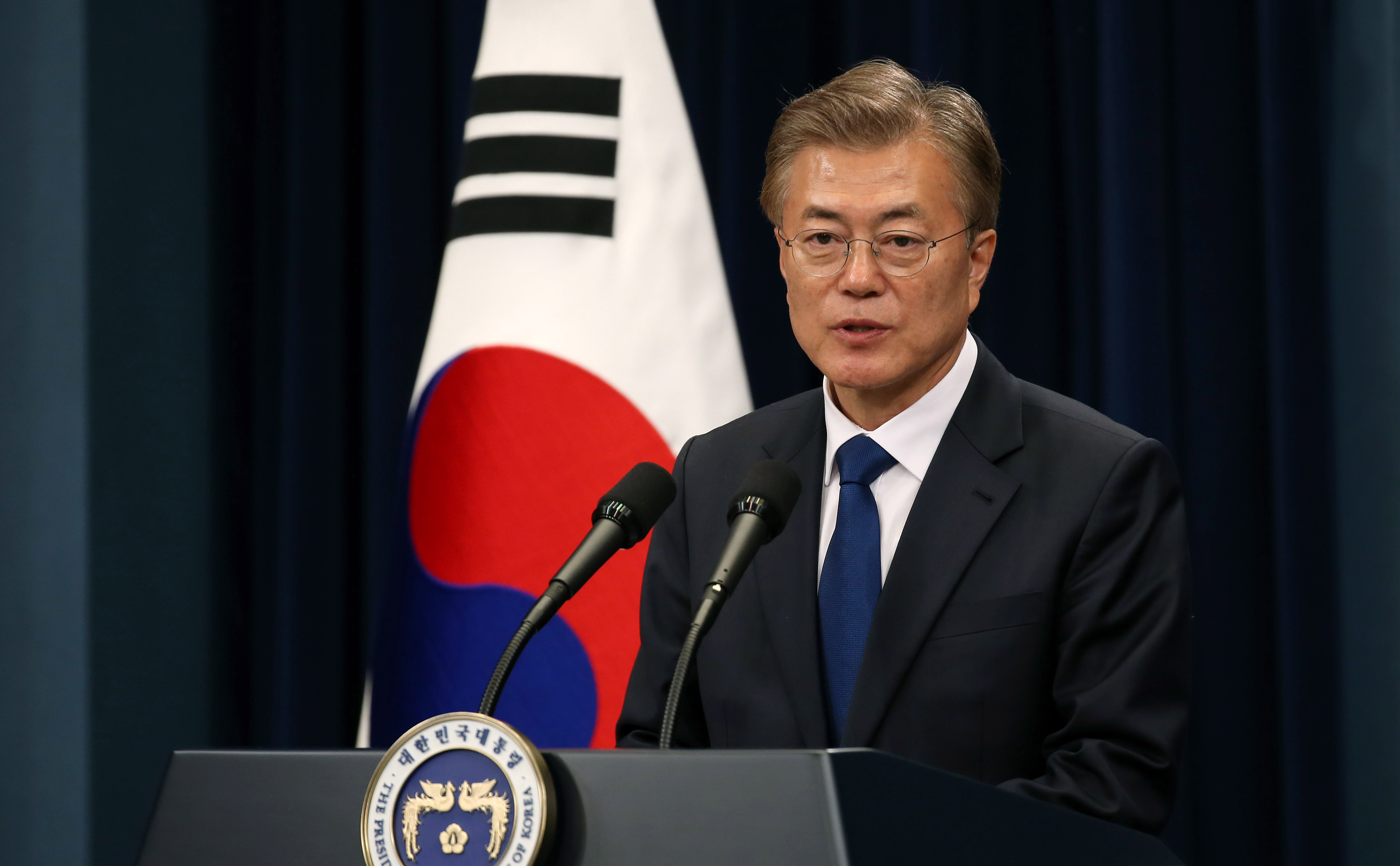This image depicts the Prime Minister of South Korea standing at a black, wooden podium equipped with two black microphones. The podium bears a round emblem featuring gold dragons and English text, symbolizing an official seal. The backdrop consists of a plain, dark navy blue curtain.

The Prime Minister, a man of Asian descent around 60 years old, has short, thinning brown hair styled in a comb over and sports round, frameless glasses. He dons a formal black suit paired with a white button-up shirt and a navy blue tie. His expression is serious as he addresses the audience, not looking at the camera. 

Behind him, a South Korean flag is visible, featuring three black horizontal stripes and a red and blue yin-yang symbol within a white background. The setting indicates a high-ranking official event, possibly a press conference or important political address.